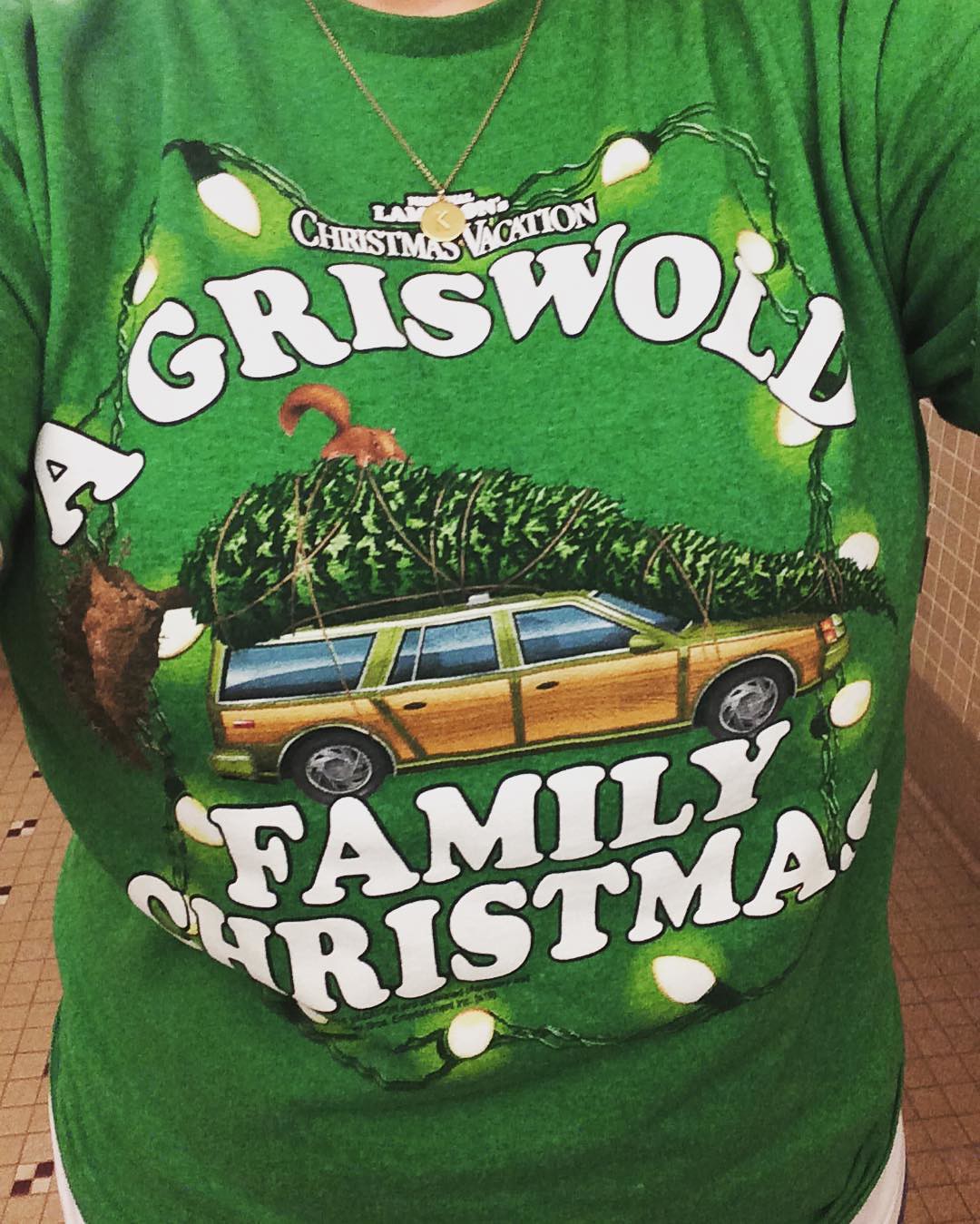This is a tall, rectangular photograph taken indoors, depicting a person wearing a visually striking green sweatshirt. Only the torso is visible, suggesting the image was likely captured by the individual holding the camera. The sweatshirt prominently features a graphic illustration central to the design: a green station wagon with wood paneling, driving towards the right, carrying an elongated Christmas tree on its roof. Notably, there is a head with a brown ponytail atop the tree, adding a whimsical touch. 

Encircling the station wagon graphic is a festive string of old-style, large Christmas bulbs, creating a nostalgic feel with two to three lights on the top, bottom, and sides. The text on the sweatshirt, displayed in bright white font, reads "National Lampoon's Christmas Vacation, a Griswold family Christmas." This design element is a clear reference to the beloved holiday movie, "Christmas Vacation," which adds a sentimental and iconic flair to the garment. The strong, appealing green color of the sweatshirt enhances its festive and nostalgic appeal, evoking memories of the classic film and inspiring viewers to watch it again.